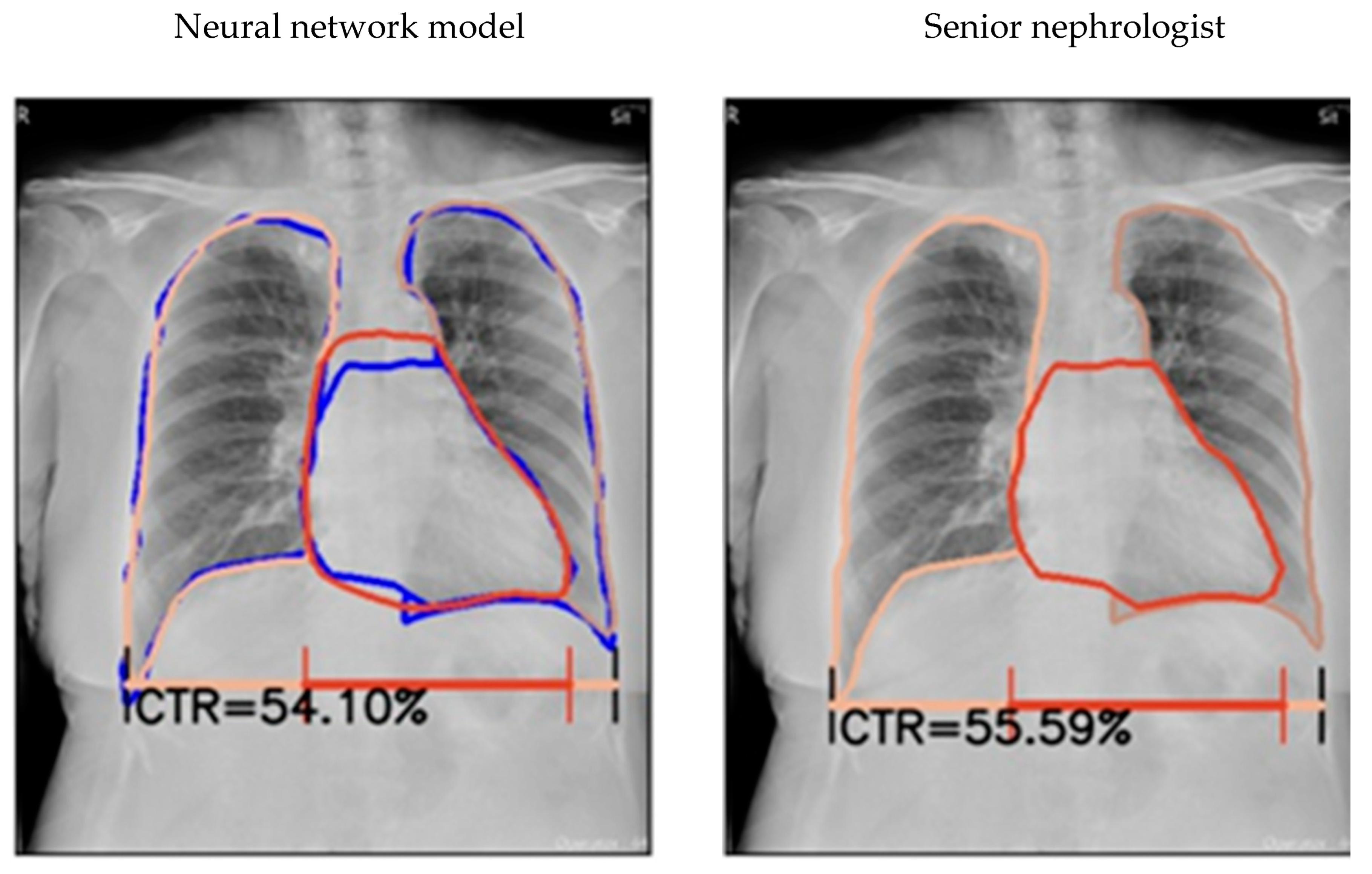This image features two side-by-side chest X-rays with digital annotations and overlaid text. The X-ray on the left is labeled "Neural Network Model," while the one on the right is labeled "Senior Nephrologist." Each X-ray displays digitally-drawn outlines around the lung regions and other areas of interest. These outlines are color-coded with blue, peach, and orange lines to denote different anatomical or pathological features. At the bottom of both X-rays, there is a measurement reading "CTR = 54.10%," indicating the cardiothoracic ratio analysis performed on the images. The detailed annotations and measurements highlight the comparative medical diagnostics between an AI model and an experienced nephrologist.